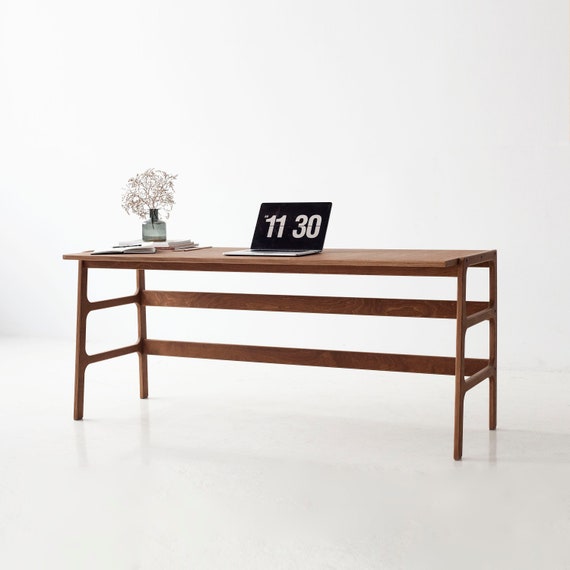The image features a meticulously arranged scene with a wooden table or desk as the focal point, set against an entirely white background, including a white floor and walls. The brown table is upright, thin, and long, characterized by its two legs at each end and two parallel wooden strips connecting its legs and back for support. The table appears to have a rectangular top with an overhanging edge at the front, while the back is flush, likely designed to be placed against a wall.

At the center of the table sits an open, silver or gray laptop displaying a black screen with a bold "1130," suggesting the time. To the left of the laptop, there is a clear glass vase containing a thin, white, bushy plant immersed in water. This side of the table is also cluttered with an open notebook, books, and a stack of papers, adding to the workspace ambiance. The overall composition of the photograph emphasizes a clean, minimalistic aesthetic while showcasing the functional workspace setup.